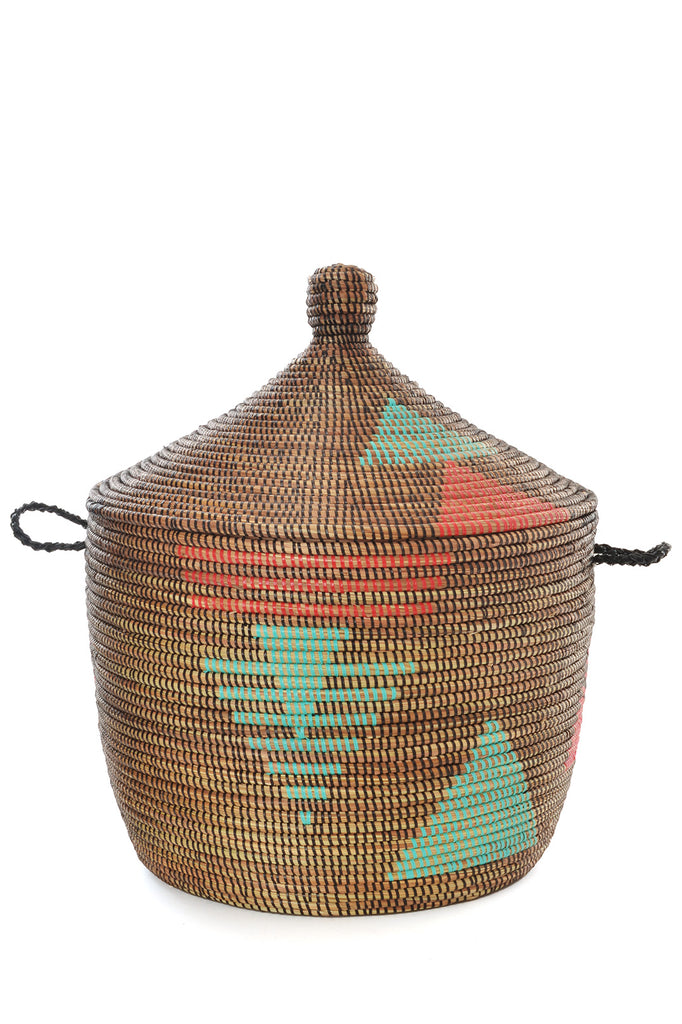This photograph captures an intricately woven, tribal hand-crafted basket, resting against a plain white background. The basket, composed of brown-reed material, features sturdy cloth rope handles positioned on either side near the top. Both the basket and its conical lid are adorned with indigenous motifs, accented with turquoise and red hues. The basket's design showcases three horizontal red lines across its upper section, above which is an upside-down turquoise triangle, layered over a larger red triangle. An additional upright turquoise triangle embellishes the lower part of the basket. The lid mirrors this symbolism with its own set of patterns: a top-most blue triangle overlaying a red triangle beneath it, culminating in a symmetrical, round-topped structure. This artifact possesses a distinctive aesthetic, likely invoking the rich cultural heritage of a Native American tribe.